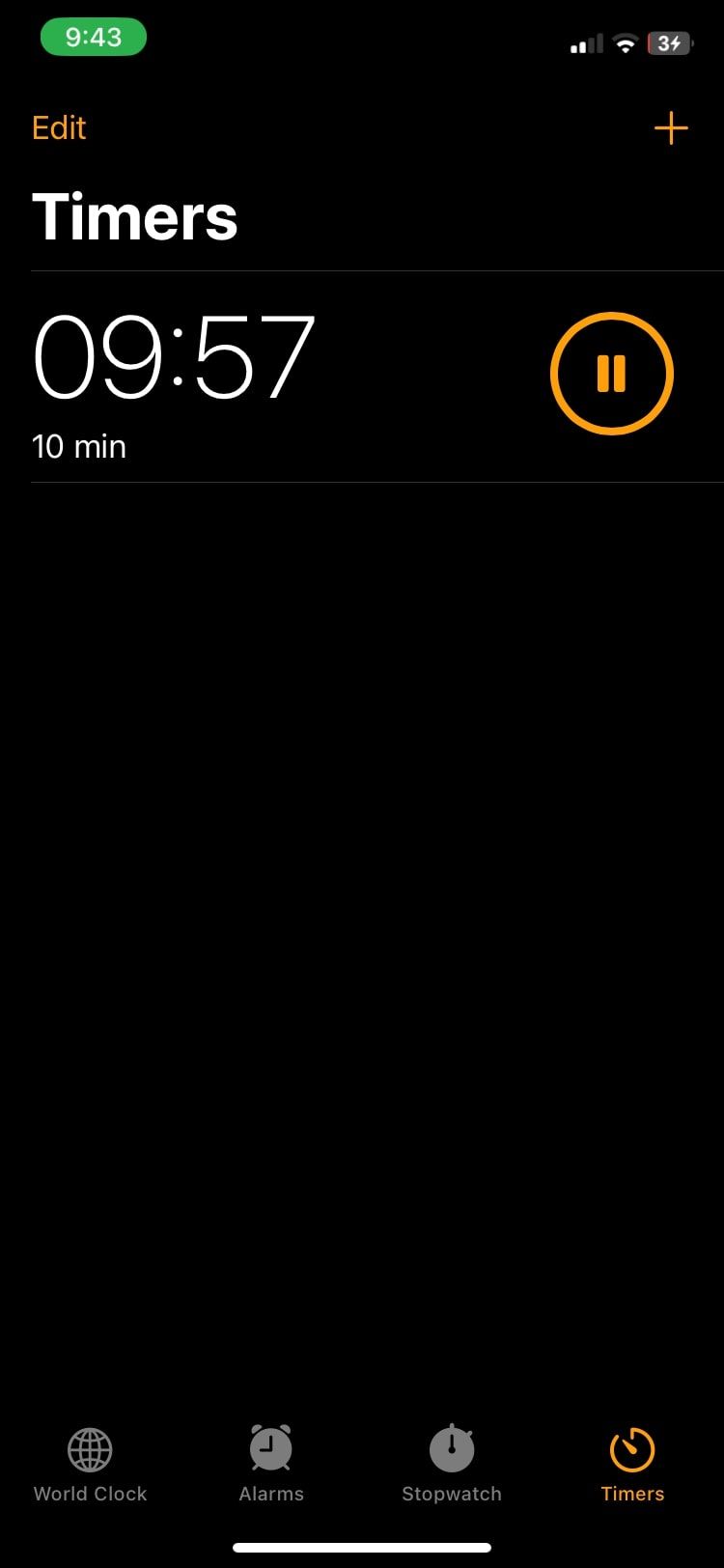This is a detailed screenshot from a smartphone. In the top right corner, the battery level is critically low at 3%, alongside two bars of cellular signal and two out of three bars of Wi-Fi signal. Located in the top left corner, the time is displayed within a green, pill-shaped icon showing "9:43." 

Beneath this, the word "Timers" appears in white text on a black background. The timer is set for 10 minutes and is currently counting down with 9 minutes and 57 seconds remaining. Adjacent to the timer, a circular pause button is visible.

At the bottom of the screen, there are four options. From left to right, they are: 
1. World Clock, represented by an icon of the Earth with latitude and longitude lines.
2. Alarms, indicated by a graphic of an old-fashioned alarm clock with two bells and a clock face showing 9 o'clock.
3. Stopwatch.
4. Timers, which is highlighted in orange.

Each option is accompanied by its respective symbol, making navigation intuitive and straightforward.